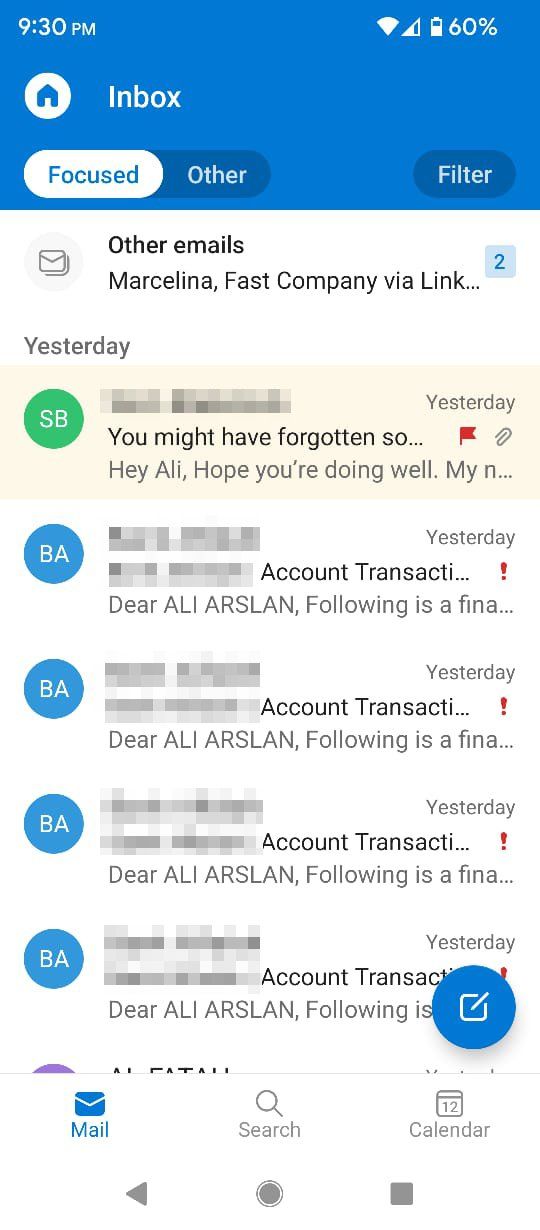Screenshot of a mobile email application interface. 

At the top, a large blue rectangle spans the width of the screen, displaying the current time on the left side and various cell phone status icons on the right. Directly beneath this, a white oval icon with a blue house symbol is positioned on the left, next to the word "Inbox" in white text. 

Below this header, there are three oval-shaped buttons lined horizontally: 
- The left button is highlighted in blue against a white background. 
- The middle button is blue with the text "Other" in light blue.
- The right button is labeled "Filter."

Under these buttons, the interface shows a list of emails. At the top left of this list, there’s an icon representing mail, followed by the bold heading "Other Emails." Below this heading, the emails are arranged in rows. 

The first section title, "Yesterday," is written in gray text, followed by a list of email previews: 
- Each email entry includes an oval icon with initials. The first email's oval is green with white "SB" initials, while the rest are blue with white "BA" initials. 
- The titles of the emails are displayed next to these icons, but the sender information is obscured for privacy. 
- The first email in the list is highlighted with a peach-colored box.

The email list continues down the screen to the bottom.